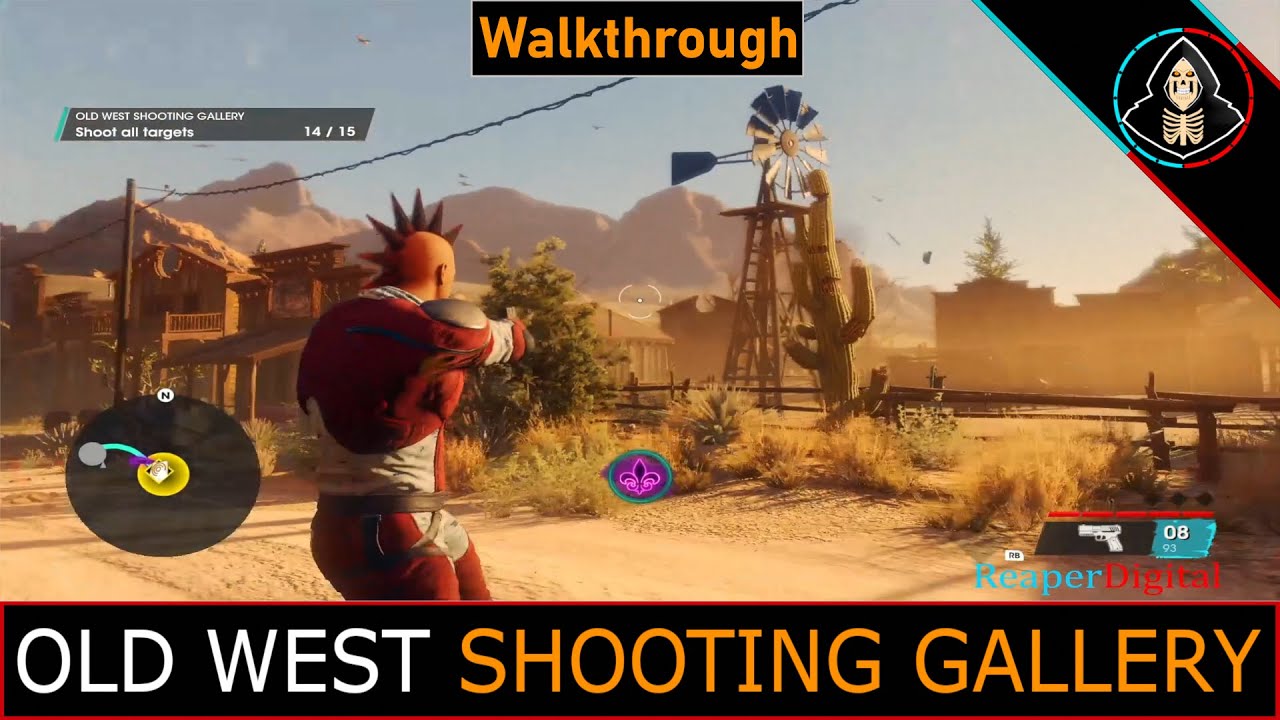The screenshot from the video game depicts an Old West-themed shooting gallery set in a desert landscape. The third-person perspective centers on a character with a spiky, brown-colored mohawk, dressed in a red and white long-sleeve shirt and matching pants. The character is aiming a gun at a blue and white windmill with a wooden base, located in the distance. The scenery includes various desert elements such as tall cactuses, shrubs, bushes, and brown mountains in the background. Sunlight shines from the upper right corner, enhancing the arid atmosphere. On-screen text includes instructions in the top left corner indicating "Shoot all targets" with a progress count of "14 out of 15." Additionally, a black banner at the bottom displays the text "Old West Shooting Gallery" in white and orange, and another black banner at the top reads "Walkthrough." The scene captures the essence of an old wooden storefront town typical of the Wild West.